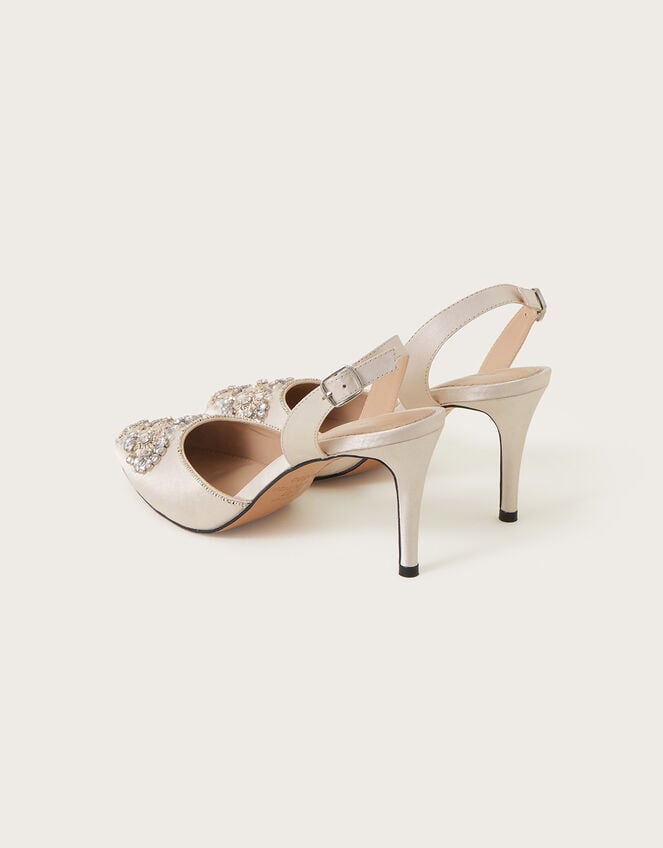This image features a pair of high-heeled women's shoes in an off-white color with several intricate details. Each shoe has a closed, rhinestone-adorned toe area, adorned with clear diamond-shaped gems that add a touch of sparkle. The shoes feature a strap around the ankle that resembles a small belt, complete with a silver clasp. The interior and the sole of the shoes are a light tan or brown leather, offering a subtle contrast to the exterior. The back of the heel is distinguished by a black tip. There is also a slight black border around the front opening of the shoes. The entire setting is on a white background, highlighting the elegance and detailed design of the high heels.